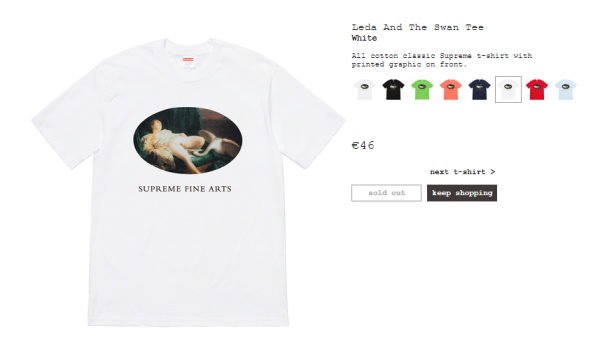This image is a screenshot of a product page from a website, displayed against a white background. Dominantly positioned on the left side is a photograph of a white t-shirt. The t-shirt features a white tag protruding from the neckline with an indiscernible red rectangle and white text due to blurriness. Adorning the chest of the shirt is an oval-shaped graphic depicting a man reclining in a chair, accompanied by an animal resembling an elephant on the right side. Below this image, in black serif text, the phrase "SUPREME FINE ARTS" is boldly displayed in all caps.

On the right side, at the top, serif script-type text reads "Leda and the Swan Tree White." Beneath this heading, a smaller font describes the item as an "All cotton classic Supreme t-shirt with printed graphic on front." A series of thumbnail images of the same t-shirt in various colors is aligned horizontally: white, black, green, pink, dark blue, white, red, and light blue.

Further down on the left side, aligned with the main text, the price is listed as "46 euros." Slightly to the right, a smaller text with an arrow indicates "Next t-shirt." Below, two buttons facilitate user interaction: a white button with a medium gray border and text proclaiming "Sold Out" on the left, and a black button with white text saying "Keep Shopping" on the right.